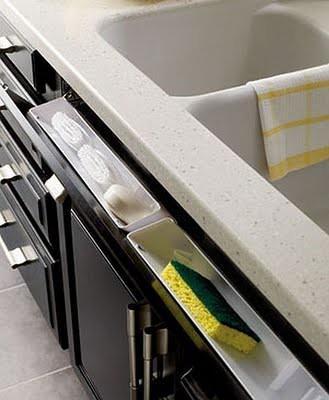The image depicts a well-organized kitchen island featuring a stainless steel sink positioned centrally on a pristine white countertop. On the right side of the sink, there are plastic storage bins in the undercarriage, one of which holds a yellow and blue sponge. The left side of the sink is equipped with soaps and towels, neatly arranged for easy access. Draped over the middle of the sink is a white and yellow cloth. Below the countertop, black drawers with sleek handles provide additional storage options, including a swing-open drawer directly beneath the sink. The bottom area showcases white bins with fold-open compartments, offering practical storage cubbies. The flooring underneath the kitchen island is tiled, creating a clean and polished look. Metal bars on the left side of the island are designed to facilitate the opening of some drawers, enhancing both functionality and design.